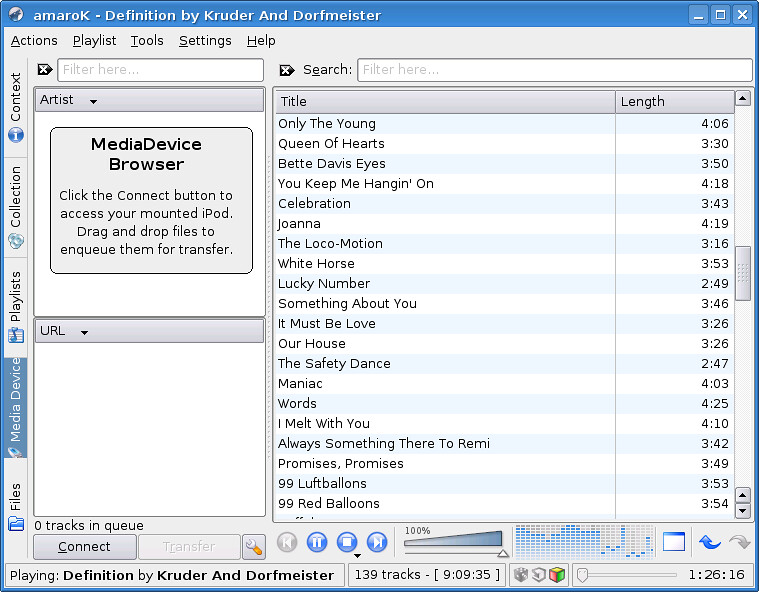The image is a synthesized screenshot of an Amarok media player interface, showcasing a detailed and organized display of a playlist. The interface features a blue lining with control icons for minimize, windowed, and close at the top right. Prominently, the title bar reads "Amarok, definition by Kruder and Dorfmeister." Along the left side, there are two distinguished white boxes labeled "artist" and "URL," with instructions to connect and manage a mounted iPod in the "artist" box, set against a gray background with black text.

On the right side, a comprehensive list of song titles is displayed in black text, including tracks such as "Only the Young," "Queen of Hearts," "Betty Davis Eyes," "You Keep Me Hanging On," "Celebration," "Joanna," "The Locomotion," "White Horse," "Lucky Number," "Something About You," "It Must Be Love," "Our House," "The Safety Dance," "Maniac," "Words," "I Melt With You," "Always Something There to Remind Me," "Promises Promises," "99 Luftballons," and "99 Red Balloons." Below the song list are blue and grey player controls, including pause, play buttons, and a volume slider set to maximum.

In the lower section of the interface, the Amarok player indicates that it is playing "definition by Kruder and Dorfmeister," from a collection of 139 tracks totaling 9 hours and 9 minutes. An additional toolbar below the title bar includes options such as Actions, Playlist, Tools, Settings, and Help. The player highlights the active "media device" tab on the left side, providing users with various ways to browse and interact with their music library.